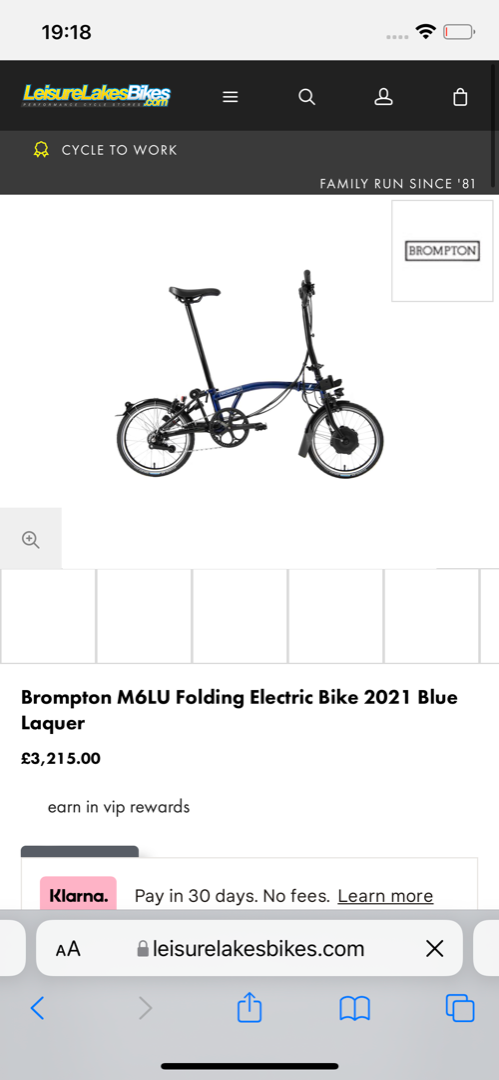The image displays the screen of a cell phone. 

- On the top left corner, the year "1918" is indicated, and on the top right, there are cellular and WiFi signal bars alongside a nearly depleted red battery icon.
  
- Below this is a black bar across the top of the screen which features the text "leisurelakesbikes.com." Above this text, there are three horizontally stacked white lines representing a menu button, a magnifying glass icon for search, a person icon likely for user account access, and a shopping bag icon.

- Underneath this black bar, there's a gray strip displaying the text: "Cycle to work family run since 1980."

- Below the gray strip is an image of a bicycle. To the right of the bicycle, the word "Brompton" is clearly visible.

- Beneath the bicycle image is a detailed description: "Brompton M6LU Folding Electric Bike 2021 - Blue Lacquer," priced at "£3215."

- The following line indicates earnings in VIP rewards.

- On the far right, there is a pink-bordered black tag with the text "Klarna" followed by a pink tab stating "Pay in 30 days. No fees. Learn more."

This composition depicts an online shopping page for a specific model of Brompton folding electric bicycle being viewed on a mobile device.